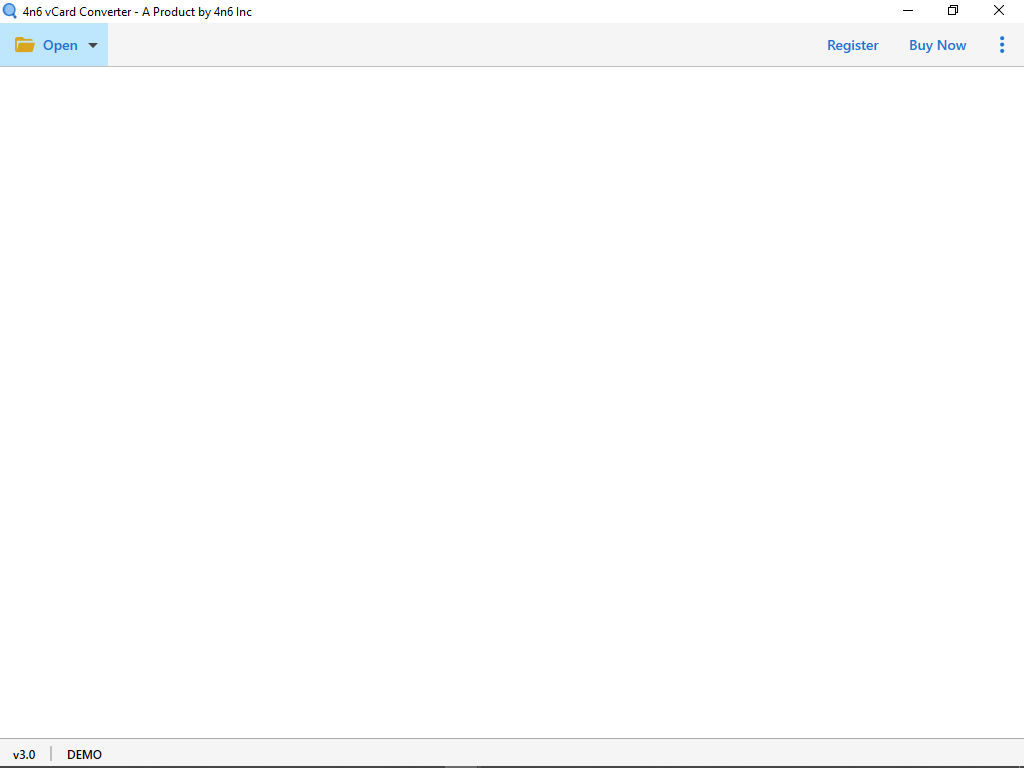The image captures a screenshot featuring the user interface of a software application. At the top of the screen, next to a magnifying glass icon used for search, the title "4n6 v-card Converter," a product by 4n6 Inc., is displayed prominently. Below this title, there's an aqua-highlighted option indicating that files can be opened, paired with buttons labeled "Register" and "Buy Now."

However, the main content area of the screen is completely empty, presenting a solid white background with no visible data or indications of any kind. At the very bottom of the screen, there's a narrow, horizontal strip that serves as a border, divided into two sections. The first section, which is relatively short, contains the text "v 3.0" in lowercase letters, followed by a vertical line, and then the text "DEMO" in all uppercase letters, spelled out as "D E M O." The remaining portion of this horizontal strip is also blank, further emphasizing the emptiness of the screen.